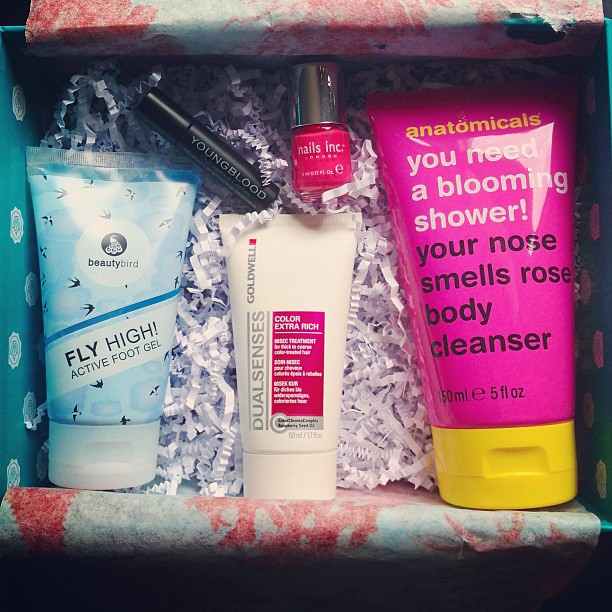This photograph showcases an open aqua blue beauty subscription box adorned with white insignias on the sides, partially visible both to the left and right. Inside, the box is packed with paper shavings for protective cushioning. Displayed within are five distinct beauty products. Dominating the scene is a large pink and yellow squeeze tube labeled "Anatomicals - You Need a Blooming Shower, Your Nose Smells Rose Body Cleanser." Adjacent is a small, hot pink nail polish bottle from "Nails Inc." A bit below is a white squeeze bottle reading "DualSenses Color Extra Rich" from Goldwell, likely a hair treatment. To its left, a blue and white bottle features "Fly High Active Foot Gel" by Beauty Bird, with a detailed design of little birds on it. Tucked above them is a slender black tube marked "Youngblood," presumably containing mascara. The arrangement of these colorful beauty products on a bed of confetti-like paper shavings creates a visually appealing and enticing presentation.